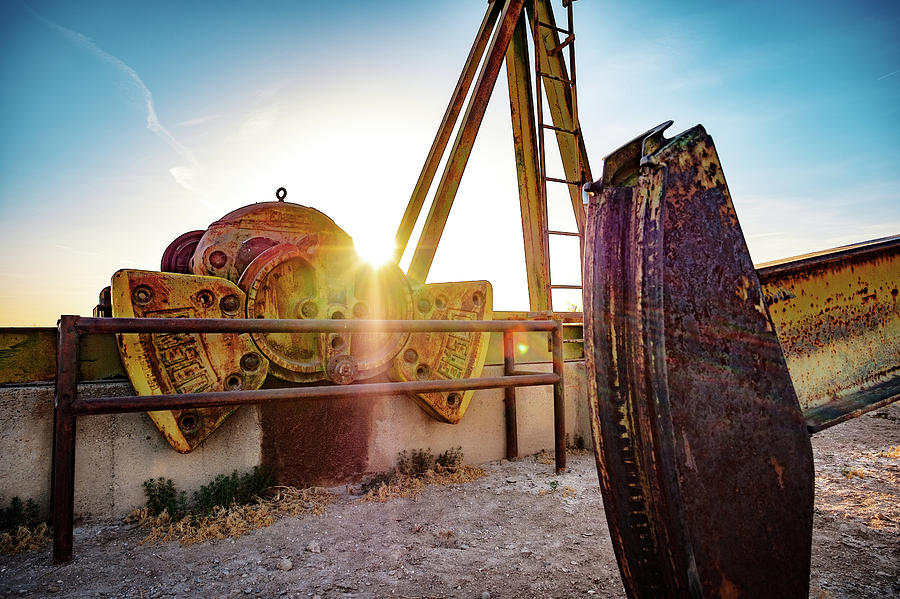The photograph depicts the head of an abandoned, heavily rusted oil drilling rig, characterized by its yellow paint that's peeling away to reveal extensive rust. This machinery, reminiscent of a bird with a beak and gears atop its head, stands out prominently. The rig's yellow-painted steel beam shaft, showing significant rust marks, is also visible. Surrounding the main machinery, there's a round shape with two wing-like sides, also painted yellow and heavily rusted. In the background, a rusty brown metal fence and a metal railing can be seen, both succumbing to corrosion. A weathered concrete wall further adds to the scene's sense of decay. The ground beneath is a mix of light brown dirt and gravel, while overhead, the bright blue sky and warm yellow sun suggest a hot day. The overall ambiance is one of industrial abandonment and severe rusting, which almost obscures the machinery's original forms and purposes.